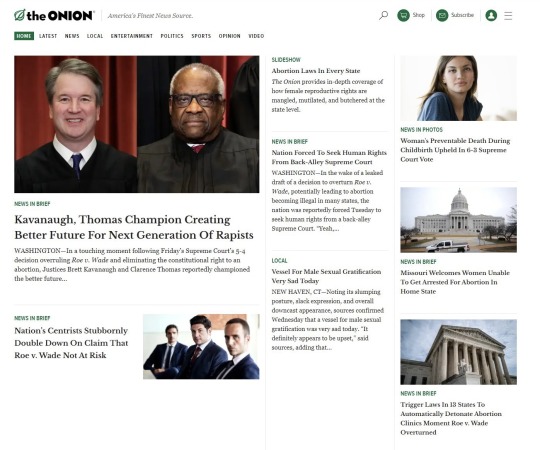This screenshot captures the homepage of The Onion's website, known for its satirical news. At the top left, you can see their iconic green onion emblem followed by their bold, black logo text, "THE ONION," with "The" in lowercase and "ONION" in uppercase. Adjacent to this logo, there is a thin gray vertical line displaying the tagline, "America's Finest News Source," in gray text. To the right, there are several interactive elements: a magnifying glass icon for search functionality, three circular buttons, and a gray hamburger menu for additional navigation options.

The top navigation bar includes nine selectable tabs labeled: Home, Latest, News, Local, Entertainment, Politics, Sports, Opinion, and Video. The "Home" tab is highlighted with a green rectangle, indicating it is the current selection.

The main content area is divided into three columns. The first column features a prominent image of Brett Kavanaugh and Clarence Thomas, accompanied by the headline, "Champions Creating a Better Future for the Next Generation of Rapists." Below this, another article appears with a photo of three men in suits.

The second column begins with a green heading, denoting a section title, followed by black text summarizing an article's content.

The third column is organized with three visual thumbnails, each accompanied by green text captions and black descriptive text beneath each image.